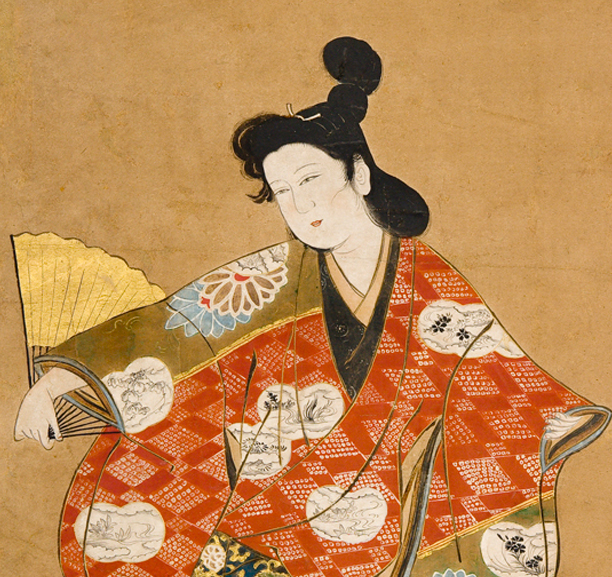This square-shaped illustration, assumed to be a drawing due to its detailed line work, features a traditional Japanese geisha as its focal point. Set against a light tan background, the graceful woman stands in the center, holding a wide-open, gold fan in one hand. Her attire is a striking blend of cultural richness, combining a loose-fitting, orange and gold kimono adorned with intricate black and white floral and diamond patterns. Subtle blue and brown flowers also embellish her left shoulder. Beneath the kimono, she wears a dark V-neck shirt, possibly black and tan. Her black hair is meticulously styled into a series of buns, both piled atop her head and at the back. Her serene, serious expression is characterized by a starkly white face, faint rosy cheeks, small dark eyes, and petite lips. She appears poised as if in a dance, gazing downward and slightly to the left, with one arm discreetly concealed within her robe.